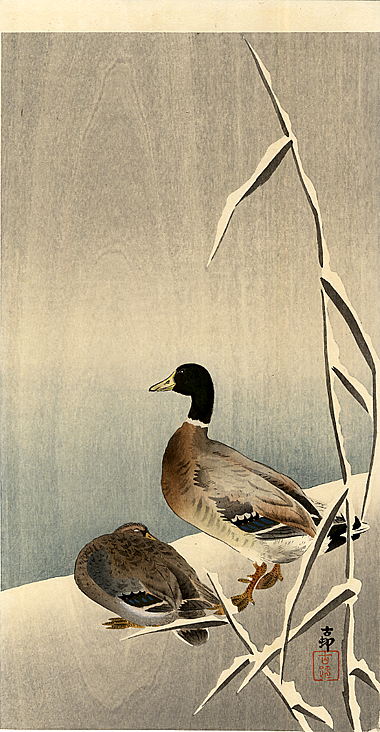This artwork is a vertical, rectangular print on wood, beautifully showcasing the natural grain through the imagery. The top of the piece features a light beige, horizontal stripe, transitioning into a gradient sky of gray to grayish white, and finally into a muted grayish-blue, suggestive of water. In the bottom right corner, sandy-colored ground supports two mallard ducks. One duck stands tall, with a striking green or black head adorned with a ring around its neck, its feathers a mix of tan, black, and white. The other duck, crouched with its head lowered, displays mostly its body. Framing this tranquil scene are two pieces of bamboo, one reaching to the top edge and the other shorter, enhancing the subtle, Asian-inspired aesthetic. The background, accented with thin, light tan grass stalks and delicate leaves, plays with shades of gray and beige, providing a serene, natural setting.